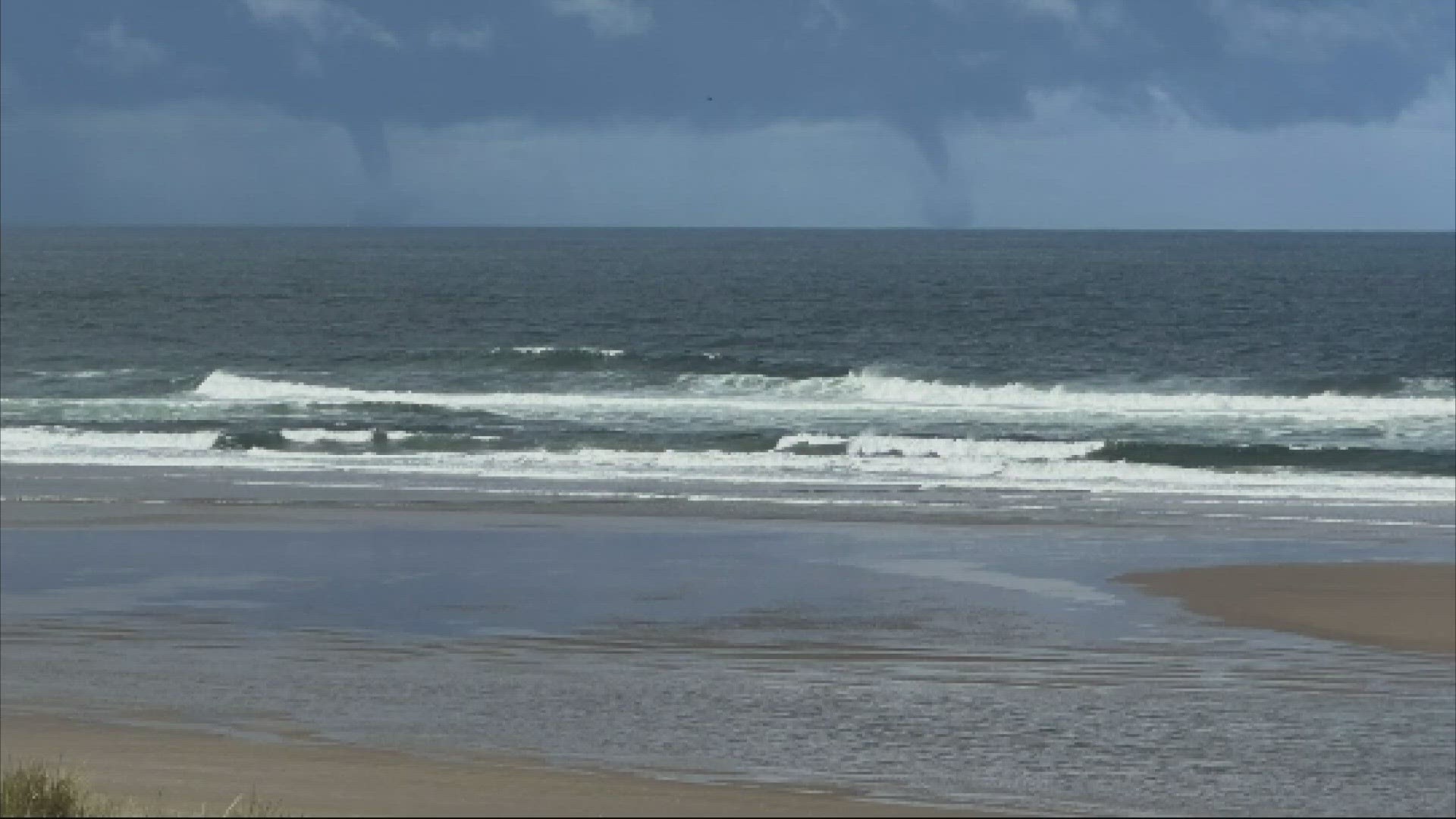This is a zoomed-in, low-quality image of a beach taken with either a cell phone or a camera. The foreground is brightly lit, showcasing the sun shining on the dark brown sand and white-capped waves washing ashore. Pockets of water are pooled in the sand, indicative of high tide. The lower corners of the image feature seaside vegetation, with a bush visible in the lower right corner and seagrass in the lower left. The water appears blue near the shore but turns dark and wavy as it moves out to sea, suggesting rough conditions. In the distance, a stark contrast is created by very dark, bluish-gray storm clouds, from which two distinct funnel clouds, or waterspouts, extend to the tumultuous ocean below. The waterspouts add to the sense of impending danger as they swirl water up into the stormy sky.